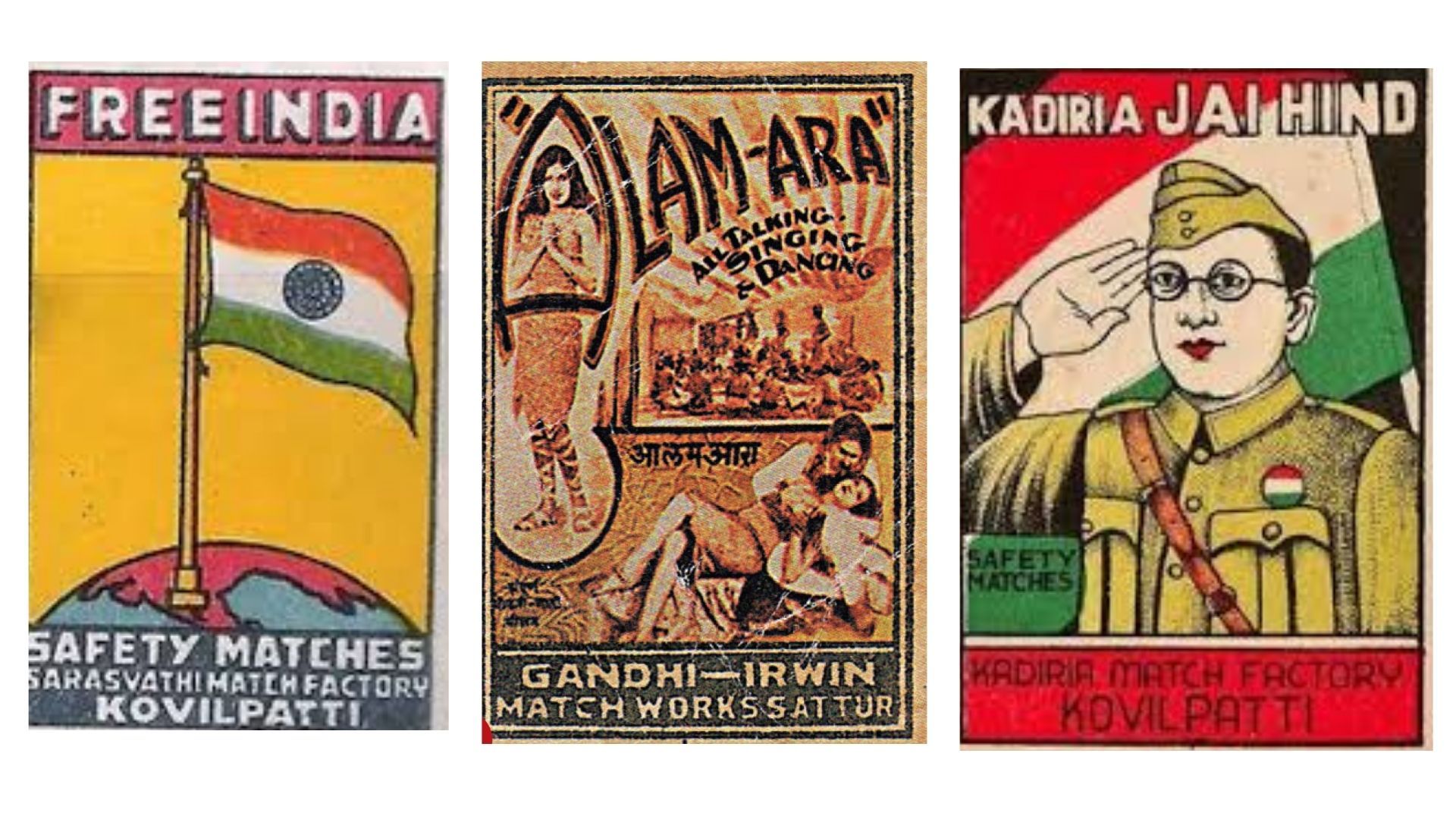The image comprises a set of three collectible matchbox covers displayed side by side, each with distinct Indian cultural and patriotic themes. 

The first cover, predominantly yellow, features the Indian flag hoisted on a gold pole atop a globe. Above the globe, white text on a red ribbon reads "Free India," while below, it states "Safety Matches Sarasvati Match Factory Cobalt Potty."

The middle cover has a tan-yellow background showcasing a scene with an Indian woman dancing and a couple seated on the ground, with the man clasping the woman from behind. The black text at the top reads "The Vamara, All Talking Singing and Dancing," and the yellow text at the bottom mentions "Gandhi Erwin Matchwork Satur."

The final cover depicts a cartoonish Indian soldier saluting in front of the national flag. The soldier, dressed in a green uniform with a black sash and wearing glasses, is portrayed with striking red lips. At the top, white text on a red ribbon spells out "Kaderia Jai Hind," and at the bottom, black text against a red ribbon says "Kaderia Match Factory Cobalt Potty."